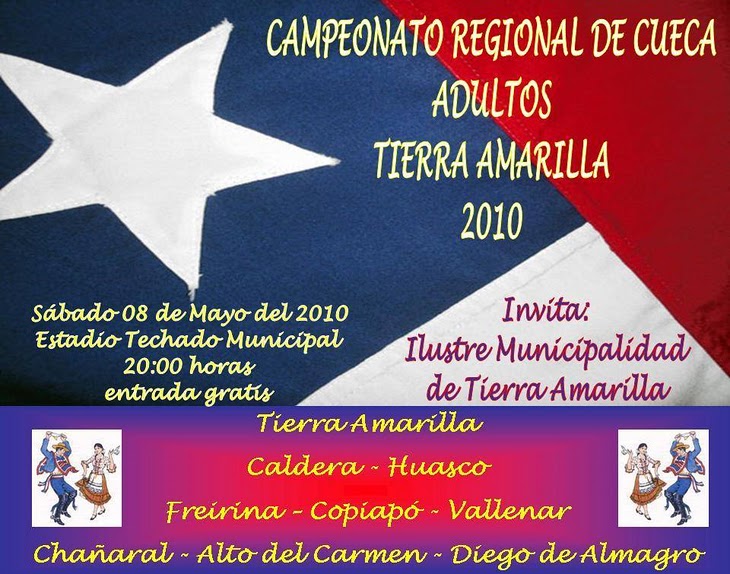This image appears to be an advertisement for a regional event, likely a festival or dance competition, emphasizing both its cultural significance and detailed schedule. The upper left-hand corner displays a large white star set against a blue background, reminiscent of a flag. Adjacent to this, the upper portion of the image contains bold, yellow text in Spanish, reading "CAMPEONATO REGIONAL DE CUECA," followed by "ADULTOS," "TIERRA AMARILLA," and "2010." The flag motif continues with a red triangle in the upper right-hand corner and a white triangle featuring additional text. Below the white star, further details are provided in Spanish, stating "SABADO 08 DE MAYO DEL 2010," "ESTADIO TECADO MUNICIPAL," "20:00 HORAS," and "ENTRADA GRATIS." The invitation is extended by "ILUSTRE MUNICIPALIDAD DE TIERRA AMARILLA," positioned over the white part of the flag. The bottom half of the poster integrates colorful patterns with a purple, pink, and orange background. Centered text lists locations such as "Tierra Amarilla," "Caldera-Huasco," "Freirina-Copiapo-Vallenar," and "Chanaral-Alto del Carmen-Diego de Almargo," in yellow letters. Framing this are small, cartoon-style images of a male and female dancer on each side, both dressed in traditional Mexican outfits, with the woman playing an instrument and the man wearing a hat and matching attire.